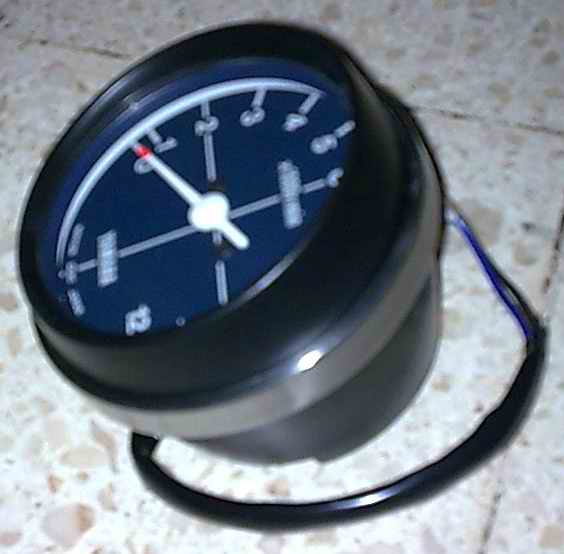The photograph features an outdoor thermometer placed on a marbled tile floor. The background consists of white tiles adorned with light brown and dark brown specks, arranged in a square pattern, though the background is noticeably blurry. 

In the bottom right-hand corner, a blue strap made of what appears to be vinyl rests against the floor. This strap is attached to a dark blue metal structure that is accented by a silver rim at the top. Inside this silver rim is a dark blue circular object, which could be made of either wood or hard plastic. 

The face of this dark blue circle is painted sky blue, and has white numerals printed around its edge, marking measurements from zero to six. A small hand with a red tip points to the zero. The precise function of this instrument is unclear.